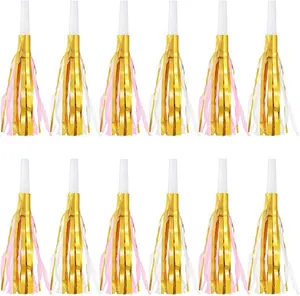The image depicts a set of 12 decorative party blowers, commonly used as party favors for events like New Year's Eve or birthdays. These blowers are arranged in two rows of six, meticulously aligned next to each other against a white background. Each blower consists of a white plastic mouthpiece at the tip, transitioning into a golden body adorned with metallic streamers. The streamers alternate in color, featuring gold interspersed with either light pink or white strands, creating a pattern of gold-pink and gold-white combinations. These blowers, when used, are intended to produce noise and create a festive atmosphere, although these particular ones appear to focus more on the visual appeal with their tinsel decorations rather than the traditional unfurling and noise-making function.